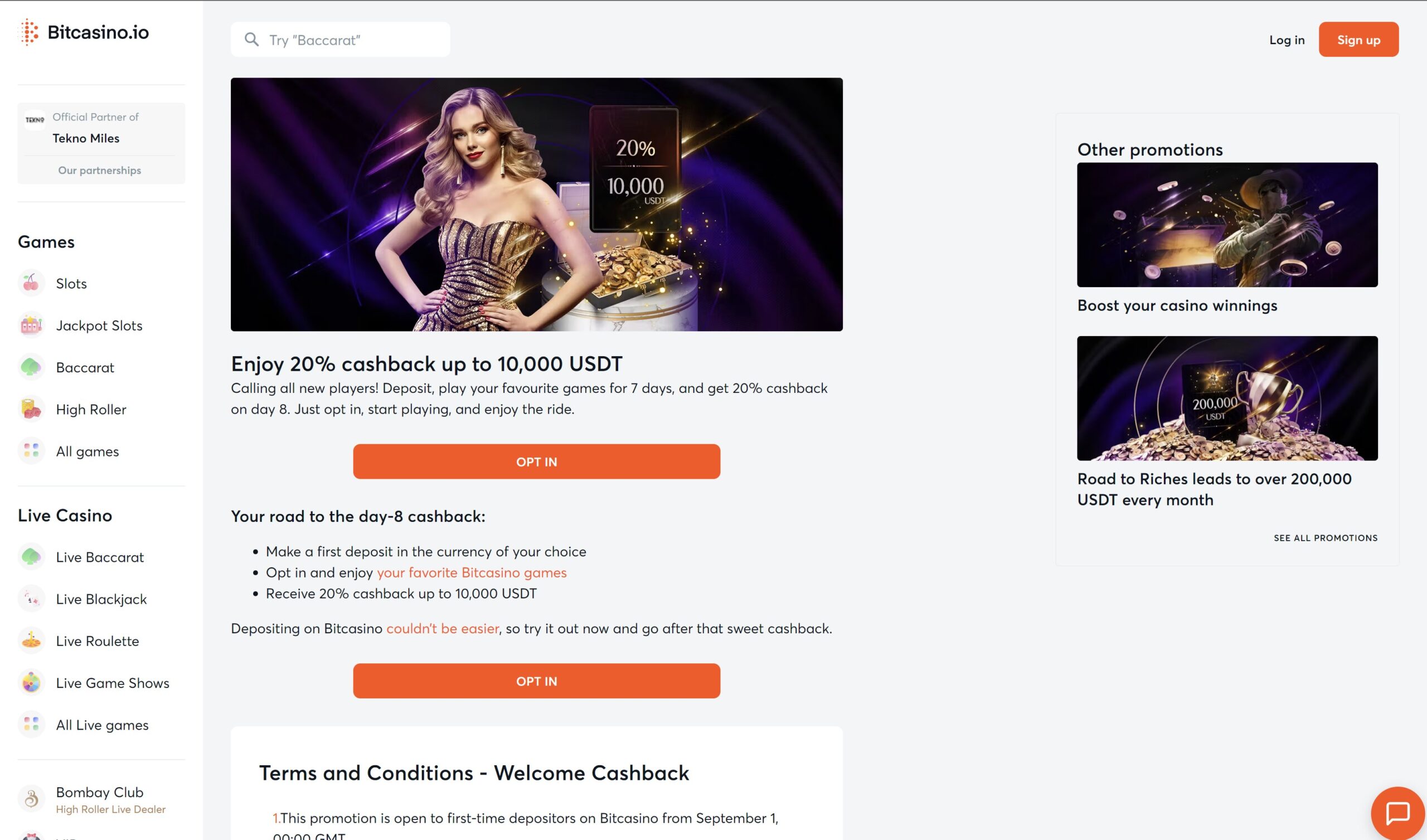This screen capture showcases the homepage of the BitCasino.io application. 

In the upper left-hand corner, the BitCasino logo is prominently displayed, followed by the website name, "BitCasino.io." Adjacent to this, a search bar prompts users with the text "Try Baccarat." 

The upper right-hand corner features two buttons for user account management: a "Login" button and an eye-catching orange "Sign-Up" button.

On the far left side of the screen, a vertical navigation column categorizes various gaming options, ranging from "Games" and "Slots" to more specific selections like "Jackpot," "Baccarat," and "High Roller." The categories continue with "All Games," "Live Casino," "Live Baccarat," "Live Blackjack," "Live Roulette," "Live Game Shows," and "All Live Games."

Dominating the center of the page is a vibrant promotional image. A woman in a stunning gold and black dress stands against a striking purple background, holding a suitcase brimming with gold. Above the suitcase, bold text advertises a "20% Cashback" promotion on amounts up to "$10,000 USDT." 

Directly below this image, further details of the promotion are laid out: "Enjoy 20% cashback on up to $10,000 USDT, calling all new players!" Participants are instructed to "deposit, play your favorite games for 7 days, and get 20% cash on day 8." The directive concludes with, "Just opt in, start playing, and enjoy the ride."

An enticing "Opt-In" button is positioned directly below this text, inviting users to participate in the offer.